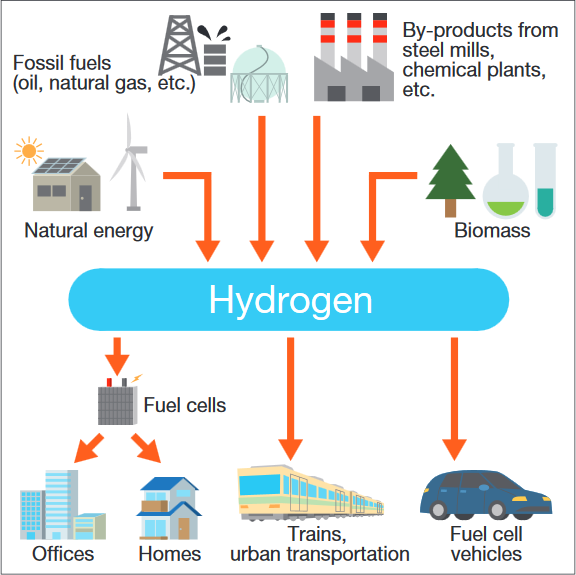The diagram is an intricate flowchart detailing the transformation of various energy sources into hydrogen and its subsequent applications. At the top, the chart features several energy sources illustrated with distinct icon-like drawings: 

1. On the far left, black text reads "Fossil Fuels (oil, natural gas, etc.)" accompanied by a dark gray oil well and a light aqua blue gas tank facility.
2. Adjacent to it, a building with three steam stacks, depicted in gray with red stripes, and the text "Byproducts from steel mills, chemical plants, etc."
3. To the right, under "Natural Energy," there's a house with solar panels and a windmill, both illustrated in light shades of gray.
4. Finally, "Biomass," illustrated with a pine tree, a green liquid-filled beaker, and a blue liquid-filled test tube.

From each of these sources, orange arrows direct downward to a central blue banner labeled "Hydrogen." This banner signifies the production of hydrogen from these diverse energy inputs.

From the hydrogen banner, further orange arrows point to various applications depicted below:

1. To the left, an arrow directs to "Fuel Cells," represented by an electrical plug icon. Below this, two arrows branch out, one leading to "Offices," and another to "Homes," each illustrated with respective building icons.
2. The central arrow flows down to "Trains, Urban Transportation," symbolized by a blue and yellow train icon.
3. On the right, another arrow points to "Fuel Cell Vehicles," depicted with a blue car icon.

The entire flowchart is set against a white background with a thin black border, making the information clear and visually organized. It effectively demonstrates the conversion of different energy sources to hydrogen and the various applications of hydrogen in powering fuel cells, urban transportation, and vehicles.